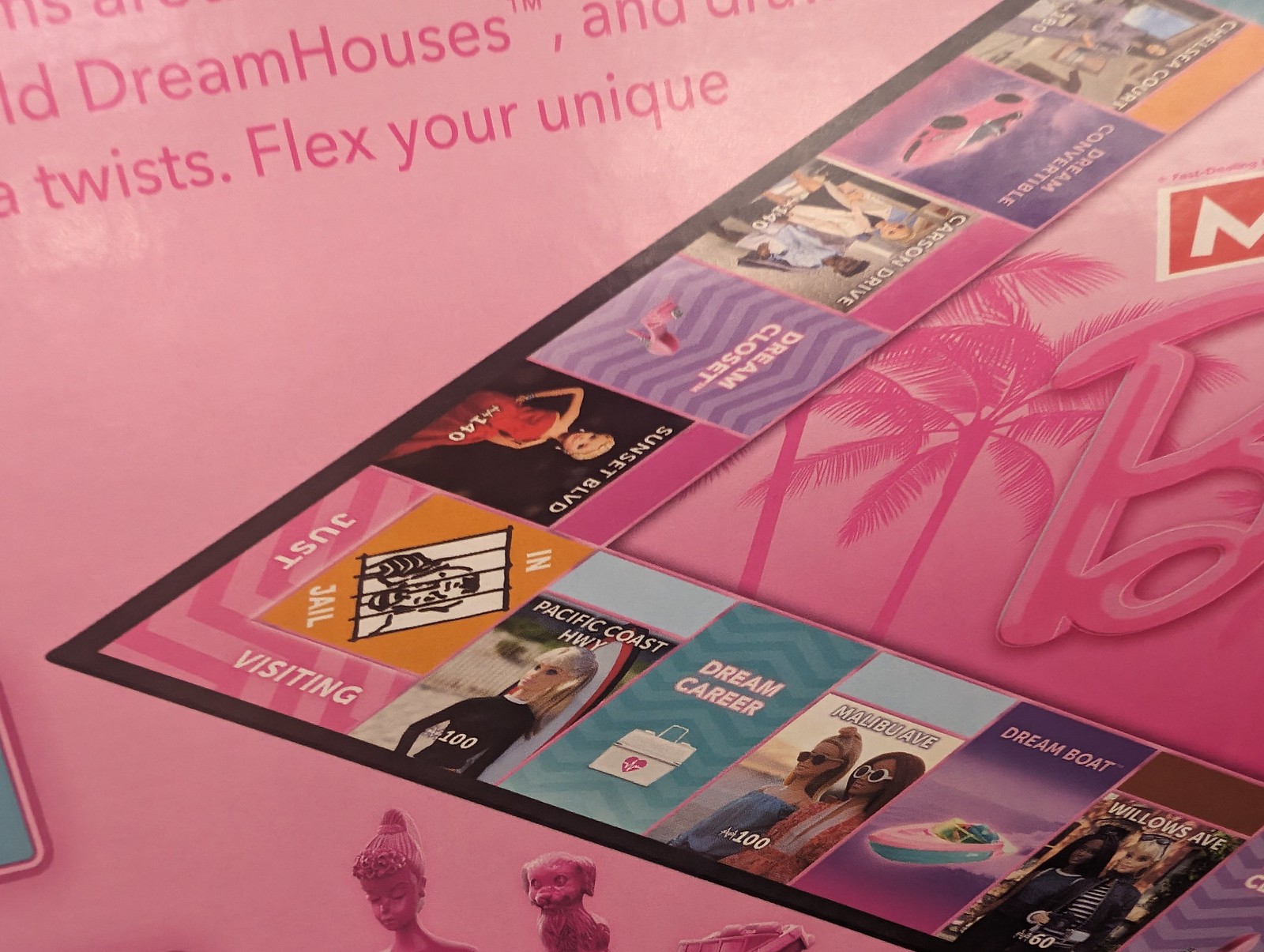The image features a partial view of a Monopoly game board, specifically themed around Barbie. Dominated by a bright pink center adorned with a stylized 'B' and flanked by palm trees, the board showcases a whimsical and glamorous setting. Starting from the bottom right corner, the properties include "Willows Avenue," "Dream Boat," "Malibu Avenue," "Dream Career," and "Pacific Coast Highway." Additionally, the corner square features the classic "Just Visiting" designation, illustrated with an image of a person behind bars and the text "In Jail." Moving upwards, the properties listed are "Sunset Boulevard" and "Dream Closet." Prominently displayed at the top of the image is the text "Dream Houses" accompanied by the phrase "Flex Your Unique." At the bottom of the image, there is a small figure of a dog and another of a girl, adding a playful touch to the overall scene.